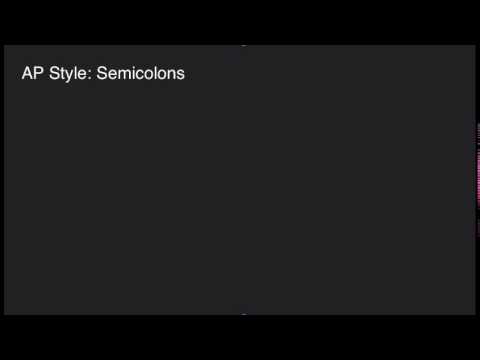The image is a horizontal rectangle with black bars occupying approximately 10% of the height on both the top and bottom, akin to letterbox formatting. The central area is dominated by a dark grey rectangle that stretches the full width of the image but stops short of touching the top and bottom black bars. This dark grey section resembles a single frame of a video, suggesting it could be either the beginning or end frame before any content plays. Within this grey rectangle, in the upper left corner, there is white block text that reads "AP Style: Semicolons," with "AP" capitalized, as well as the "S" in both "Style" and "Semicolons." Additionally, there are very light specks centered at the top and bottom of the grey rectangle. There are no other objects, characters, or elements in the image, emphasizing the text.